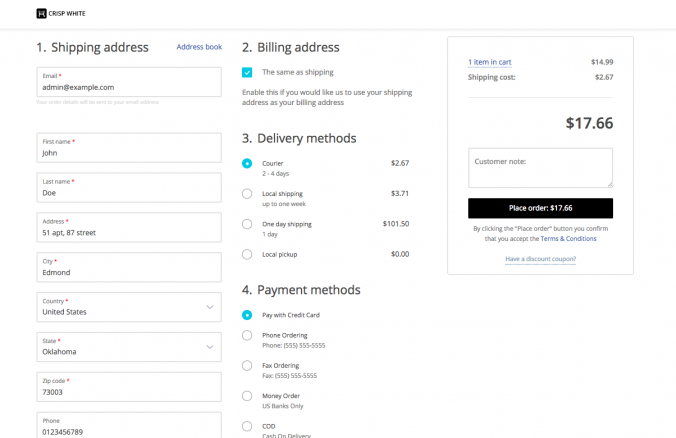This image displays a screenshot from a webpage with the heading "Crisp White" at the top, followed by a form titled "Shipping Address." The form is partially filled out with the following example data:

- **Email:** admin@example.com (marked mandatory with a red star)
- **First Name:** John (marked mandatory with a red star)
- **Last Name:** Doe
- **Address:** 51 Apart 87 Street
- **City:** Edmond
- **Country:** United States
- **State:** Oklahoma
- **Zip Code:** 73003
- **Phone:** 0123456789 (not marked mandatory)

To the right of the shipping address form is a column labeled "Billing Address," which has a teal check mark with the option "Same as Shipping" selected.

Further down, the image details the "Delivery Methods" section, where "Courier" is selected, costing $2.67. Underneath, the "Payment Methods" section shows that the buyer has opted to "Pay with Credit Card."

The summary at the bottom of the page notes that the cart contains one item. With the added shipping costs, the total amount due is $17.66.